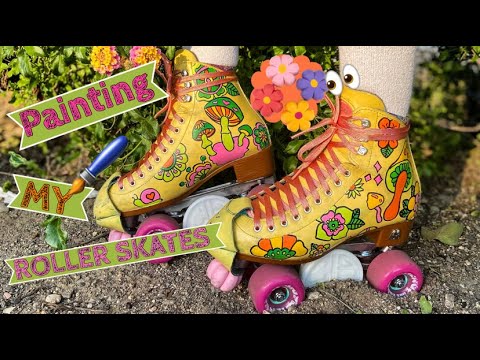The image features a vintage pair of mustard yellow roller skates adorned with brownish-orange laces that wrap around the high tops. The skates are vibrantly decorated with psychedelic mushrooms and variously colored flowers—pink, green, orange, yellow, red, and purple—strewn across their sides. The wheels of the roller skates are a bright pink. The scene appears low-resolution, possibly a video frame, with black bars at the top and bottom. The background shows the person standing in dirt with some flowers behind them. On the left side of the image, three green ribbons with white outlines display the text "painting my roller skates" in pink and orange writing. Additionally, a small paintbrush emoji with orange bristles is painting the letters "Y" and "My." The overall appearance captures a nostalgic, vibrant, and artistic aesthetic.